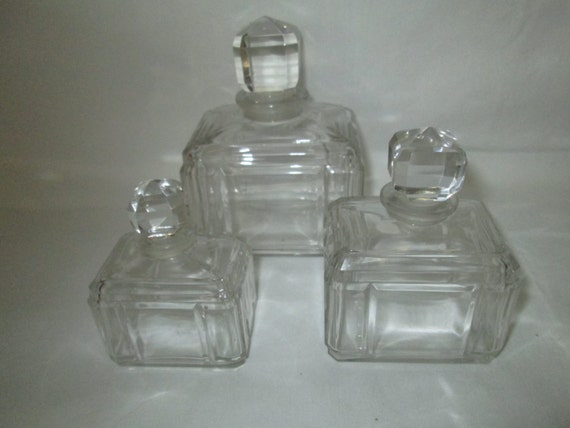The image showcases three empty, clear glass decanter bottles set against a white counter and background, which create an overall white or gray ambiance. The bottles are of varying heights but share the same rectangular shape with round tops. The tallest bottle, positioned at the back, has a square body with a round knob. The second tallest, situated on the right, is slightly smaller, also square-shaped, featuring a prism-like top. The smallest bottle, located on the left, follows the same design with a square rectangular shape and a similar prism-like top. Despite the simple, industrial-made glass design, the bottles have inlet square patterns on their sides that resemble cut crystal but are clearly mass-produced. The image captures subtle light refractions and caustic reflections on the surface, adding visual interest to the otherwise minimalistic scene.